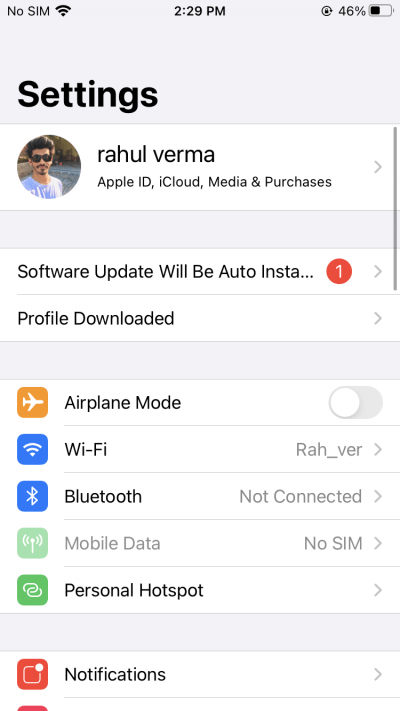**Detailed Caption of the Settings Page Screenshot:**

This screenshot captures a settings page from a cell phone. Prominently displayed in the upper left-hand corner, the screen indicates "No SIM" in black text accompanied by a Wi-Fi icon. Centered at the top, the current time is shown as 2:29 p.m., while the upper right-hand side displays a battery level of 46%.

The background of the settings page is light gray, providing a neutral backdrop for the menu options which are listed on white blocks with black text. The top of the screen prominently features the heading "Settings" in bold black letters.

Following this title, there is an icon showing a tan-skinned individual with sunglasses, a goatee, and dark hair, wearing a white t-shirt. Below this photo icon, the username "Rahoo Verma" is displayed. Further details include the options "Apple ID, iCloud, Media, and Purchases" listed underneath the username.

The first menu item visible is labeled "Software Update" with the text trailing off after "Auto Insta..." and marked with a red circle containing the number one, indicating a notification or update pending. Under this, there is a line reading "Profile Downloaded."

Following these initial items, the page displays several settings options with corresponding icons. The "Airplane Mode" is listed next, featuring a yellow square with a white airplane icon and an adjacent button showing it is turned off. Below that, "Wi-Fi" is presented with a blue square that contains Wi-Fi bars, and the Wi-Fi network name "RAH_VER" is displayed at the right end of this line.

Subsequently, the "Bluetooth" option is represented by the Bluetooth symbol and the word "Bluetooth," noted as "Not Connected" on the right. Other visible settings include "Mobile Data" marked as "No SIM," "Personal Hotspot," and "Notifications."